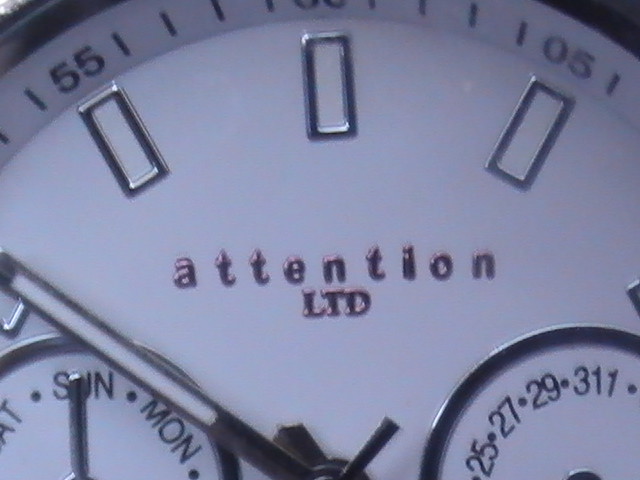This is a detailed close-up photograph of what appears to be either a clock face or a type of spin lock, reminiscent of one on a school locker. The focal point is on the top section, which features the brand name "attention" in black lowercase letters, followed by "LTD" in uppercase letters beneath. The background of the face is white, with a chrome and white inlay second minute hand positioned centrally. Along the top edge, we see three silver rectangles and additional details resembling the top markings of a clock, including numerous short lines. The numbers 55 and 05 are positioned to the left and right, respectively. In the lower left corner, there are abbreviations "SUN." and "MON." with a silver line pointing to "SUN." To the right, a circle displays the numbers 25, 27, 29, and 311. The face is embossed and contains smaller dials, likely indicating the day and date.